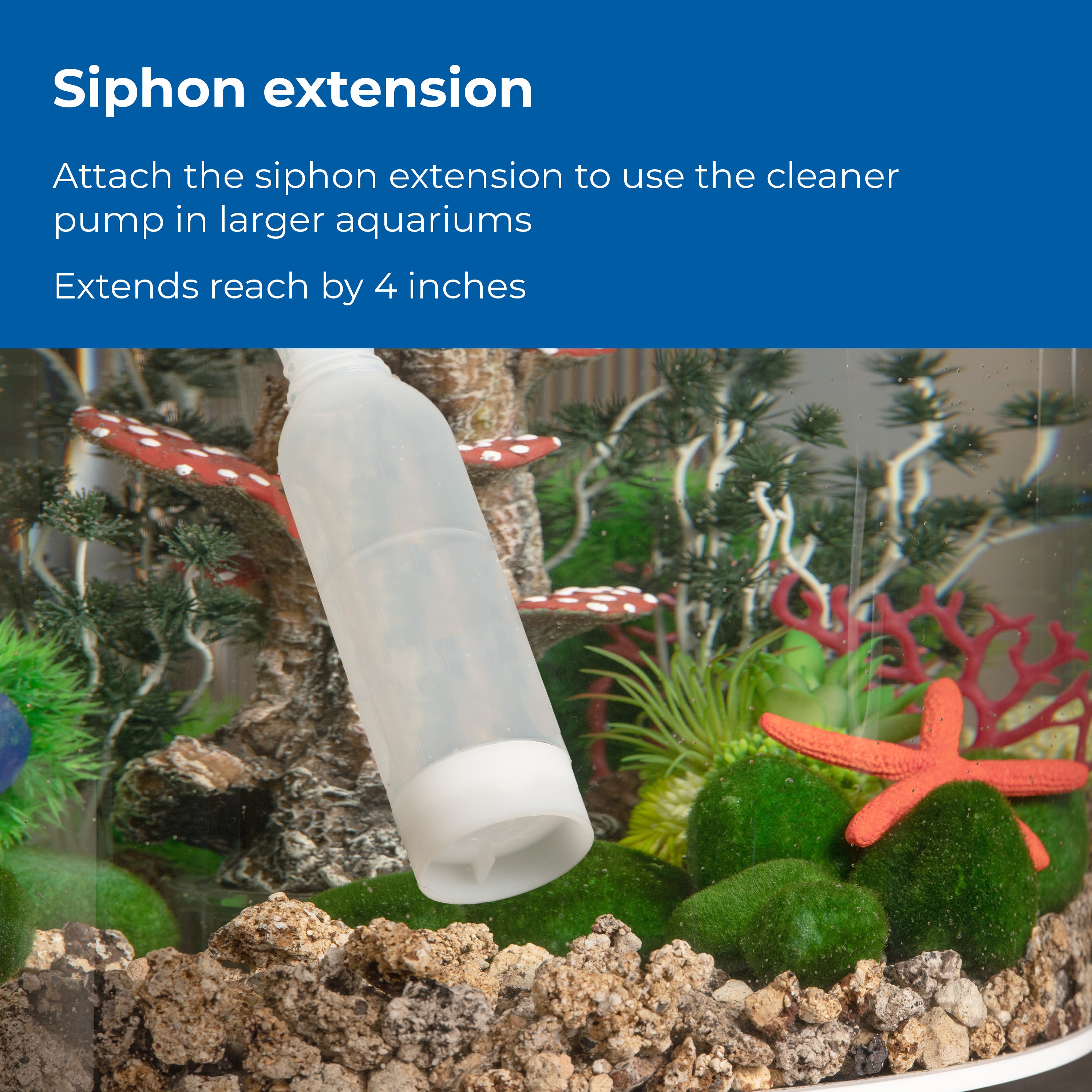This image appears to be a page from an instruction manual or informational pamphlet about aquarium maintenance. The top third of the image features a bold blue background with prominent white text that reads "Siphon Extension," followed by smaller print instructions: "Attach the siphon extension to use the cleaner pump in larger aquariums. Extends reach by four inches." Below this text, there is a detailed photo of a vibrant aquarium filled with colorful decorations. The aquarium houses artificial coral, a bright starfish, various green rocks that appear to be covered in moss, and a scattering of other decorative elements like seaweed and algae. A white cylinder, assumed to be the siphon extension, extends towards the bottom of the tank, illustrating its purpose for cleaning by siphoning out dirty water.